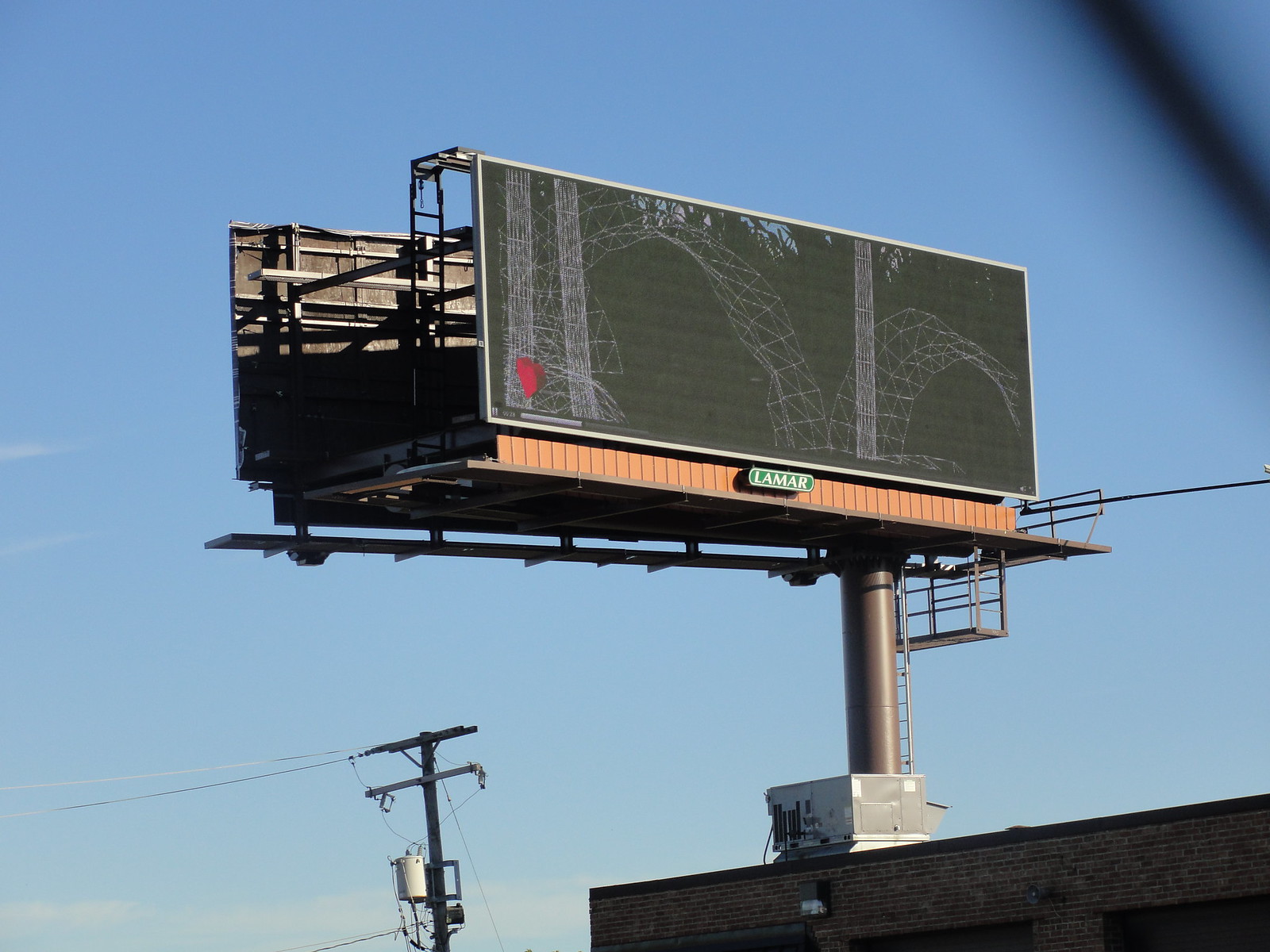This daytime photograph showcases a striking urban scene against a backdrop of clear, blue sky with thin, wispy clouds. Dominating the image is a giant double-sided billboard with a black background and an abstract white illustration, potentially depicting a bridge. Below the graphic, "Lamar" is written in green and white. Visible behind and around the billboard are intricate power lines and the upper portion of a brick building, which is topped with a distinct silver square object. The building's façade features a prominent light fixture. The back scaffolding of the billboard reveals a network of structural details. Additionally, a squat silver-white object is perched on a nearby power pole, adding to the intricate industrial aesthetic of the scene. The image is captured with exceptional clarity, allowing for easy recognition of even the smallest elements.